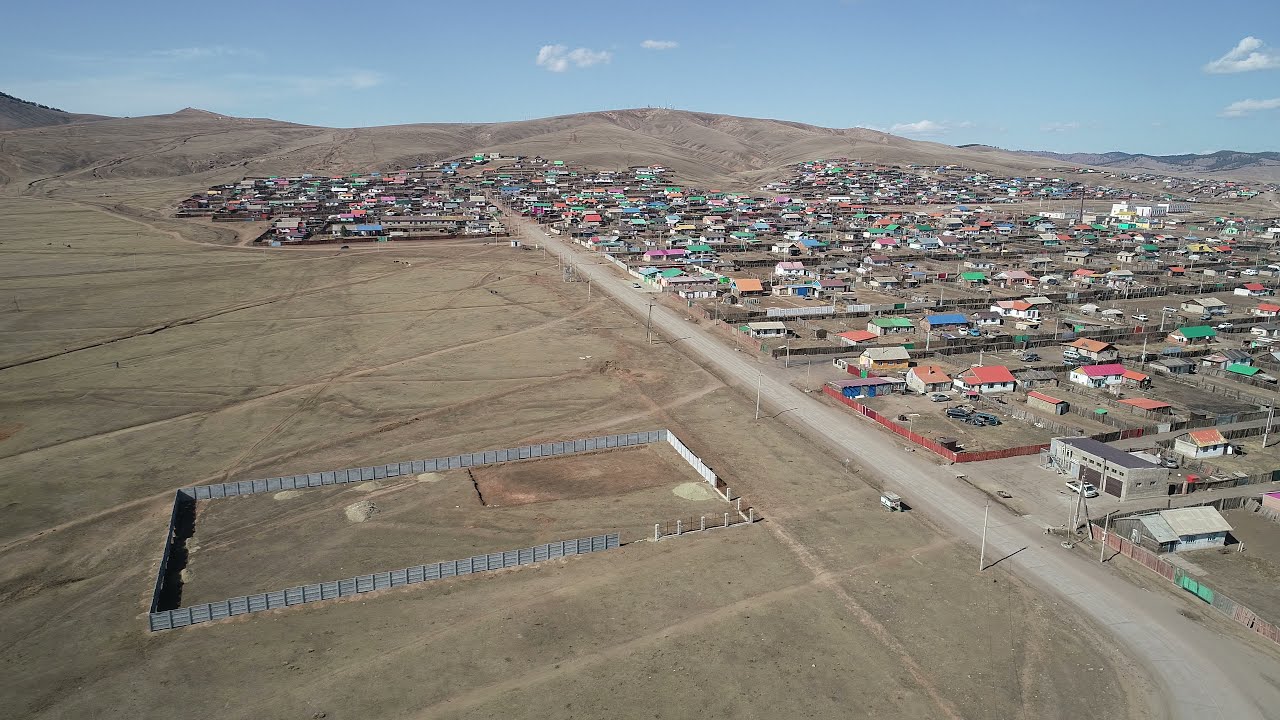This aerial image showcases the edge of a town framed by hilly terrain, possibly located in the Great Plains or the Mountain West region. The photo prominently features a road that traverses diagonally from the lower right to the upper middle, with its surface type—a mix of gravel and pavement—hard to discern. The right side of the image is dense with homes and various structures, tightly clustered together. These buildings display a palette of diverse roof colors including red, blue, green, and pink, mostly adorning white structures.

On the left side of the photo, a vast expanse of brown dirt and grassy areas is prominent, interrupted by a large rectangular plot enclosed by metal fencing, speculated to be a horse enclosure though devoid of any visible equine activity or stable. The terrain is largely bare, marked by dirt with some faint lines indicative of pathways or minor roads. 

In the photo's bottom right corner, a slightly taller building stands out—a garage or automobile service structure, recognized by its tall brown doors. Throughout the town, numerous smaller dirt roads branch off from the main road, leading to various homes and neighborhoods. As the image extends toward the horizon, the landscape transitions into rolling hills under a blue sky, sparsely dotted with clouds, devoid of trees, and interspersed with telephone or light poles along the main thoroughfare.